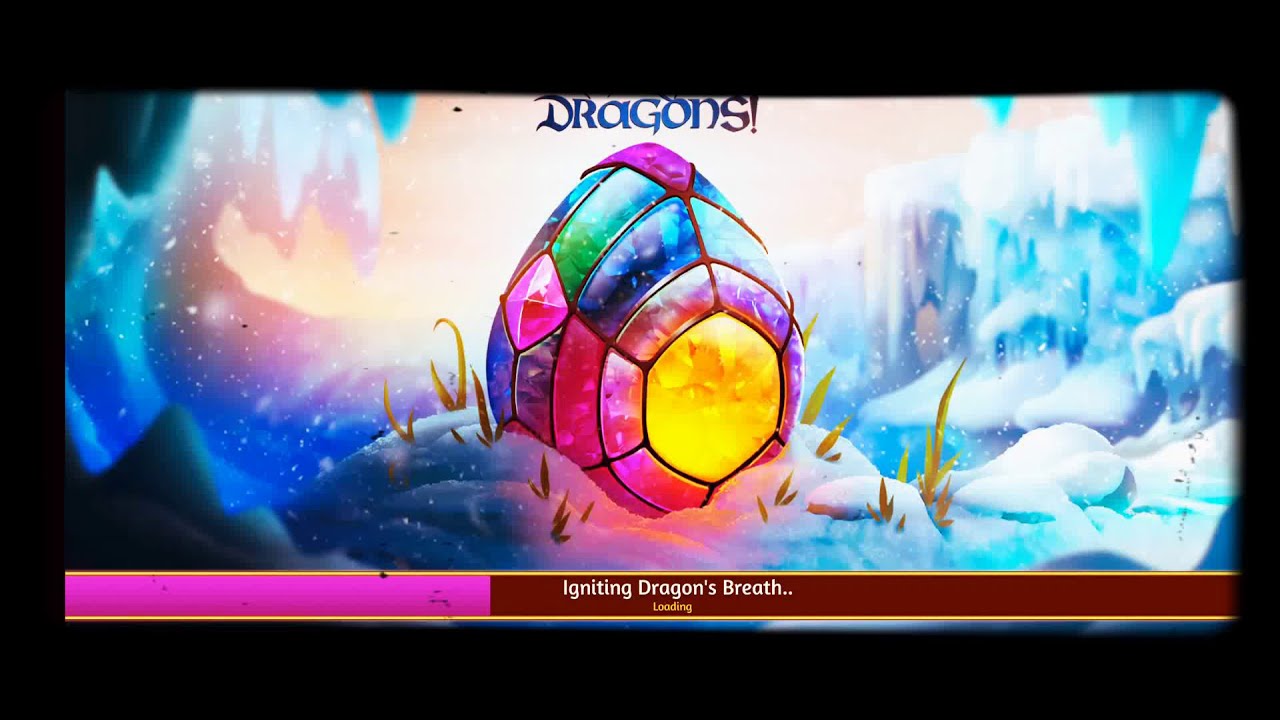This image is a vibrant and detailed screenshot from a video game, featuring a loading screen with a black border. At the top, “Dragons!” is prominently displayed in bold blue, uppercase letters, except for a lowercase "a". Below, a central focal point, resembling a crystallized, decorated egg, sits amidst a snowy landscape dotted with tufts of yellowish grass. The egg’s design is intricate, with golden yellow at its core and various rectangular stained glass panes encircling it in colors such as pink, blue, green, and purple. Diamond shapes, particularly in pink, also adorn the egg, which is encased in a terrain reminiscent of glaciers, complete with blue and white ice formations and glistening pink and white sparkles. Icicles dangle from the image's backdrop and top, enhancing the frosty wintery scene. Towards the bottom, a purple and red-striped loading bar, labeled “Igniting Dragon’s Breath, Loading,” adds to the immersive gaming experience.